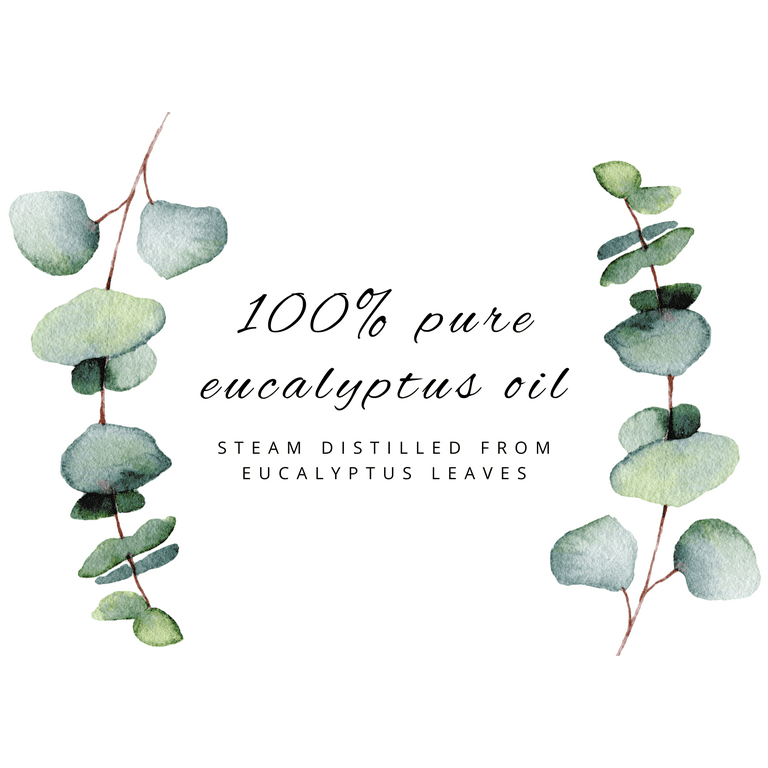The poster image features a clean white background, with two sprigs of eucalyptus leaves on either side. The sprig on the left points downwards while the one on the right points upwards, with both stems being dark brown. The leaves, which are not very pointed but rather rounded and heart-shaped, vary in color from dark green to blue-grey and appear opposite each other on the stems, though not consistently. In the center of the image, black text reads "100% pure eucalyptus oil" in a script-like, lowercase font with separation between each letter. Below it, in smaller, all-caps text, it states, "steam distilled from eucalyptus leaves."